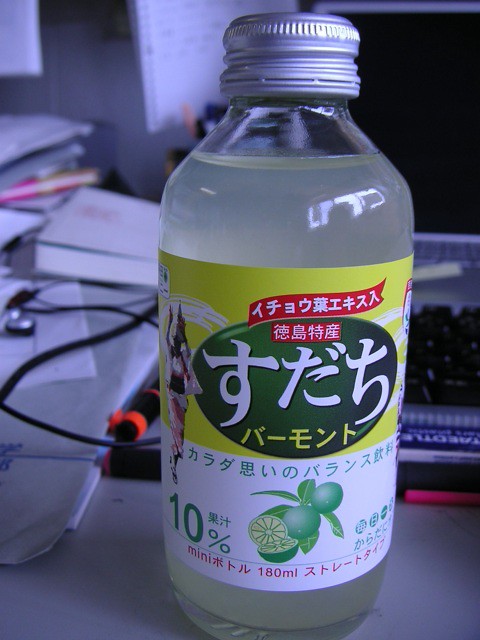The image showcases a cluttered office setting with a prominent white desk cluttered with various items, and a white cabinet and some books and papers in the background. On the desk, there's a close-up shot of a transparent glass bottle of juice with a silver metal screw cap. The bottle features a yellow and white label, with Japanese hiragana, katakana, and kanji characters. The label includes green text indicating "10%" and "mini 180 ml." The design on the label features a picture of a woman in pink and white apparel on the left side, a large lime cut in half at the bottom, and two whole limes on a branch. Additionally, there is a black keyboard, a black cable, a pink and black pen, an orange and black pen scattered on the right side of the desk.